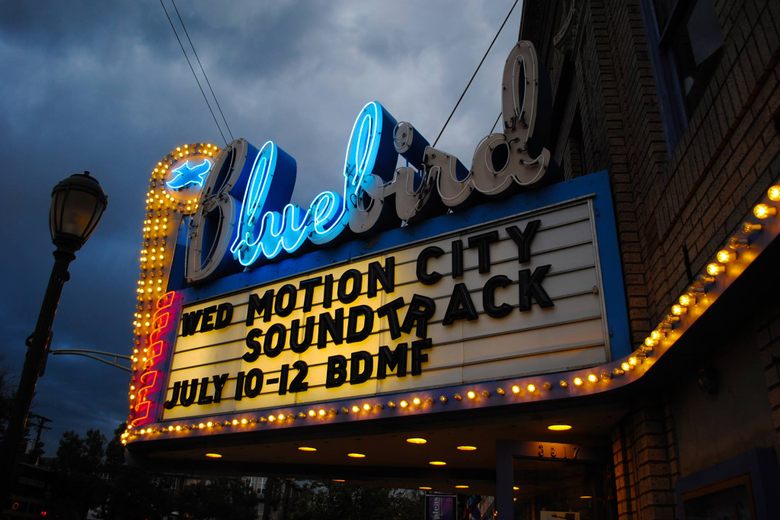In this outdoor photograph taken at twilight, we see the exterior of an aging theater. The theater's facade is constructed with timeworn bricks, hinting at its historical character. A marquee-style sign hangs prominently on an awning, providing shelter for patrons below. The marquee sign announces "Wednesday Motion City Soundtrack, July 10th - 12th, BDMF," though the letters "T" and "R" are precariously hanging from their mounts. Above the marquee, a partially illuminated blue neon sign intended to read "Blue Bird" fails to do so entirely, as most of the letters are burnt out. Instead, only "LUL" is visible since the "B"s, "I," "R," and "D" are not lit. Despite the general disrepair, a small neon bird to the left of the sign remains lit. Additionally, a series of carnival-style bulbs beneath the sign, where half are burnt out, cast a dim, uneven light. The image captures a dark, brooding atmosphere with storm clouds gathering on the horizon, suggesting an impending rainstorm.